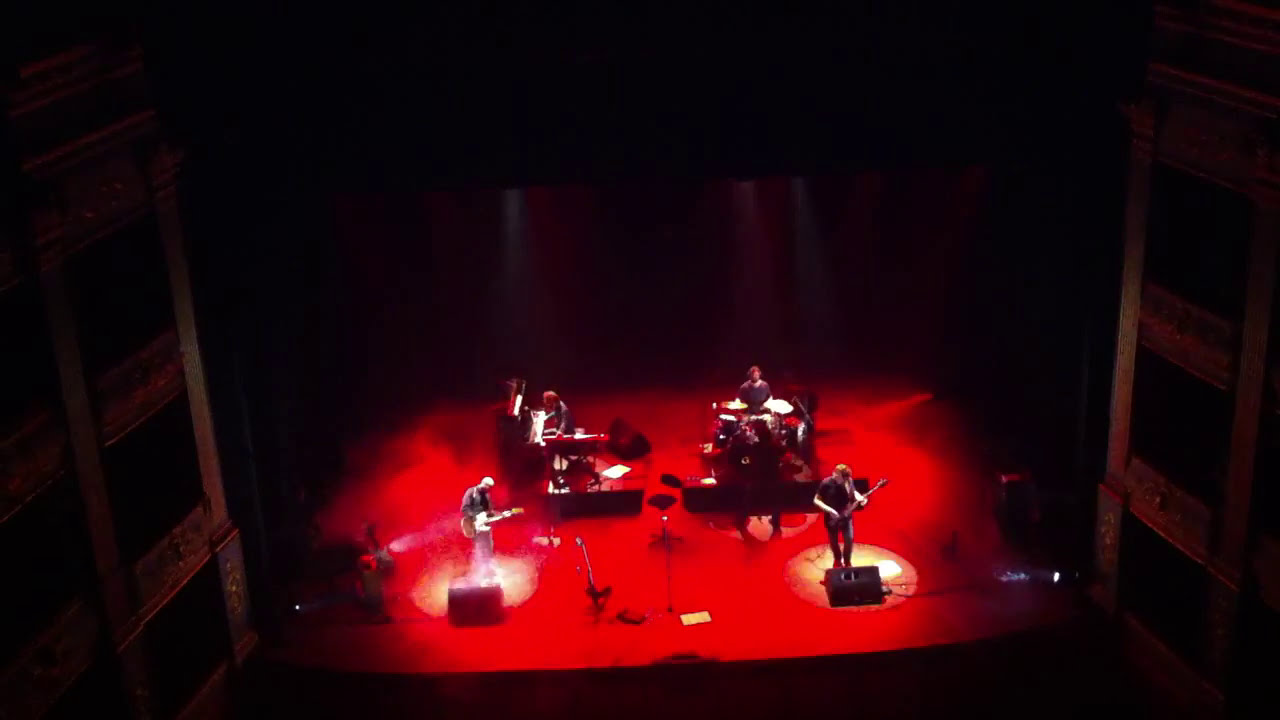This photograph captures an overhead view of a dimly lit indoor stage featuring a band of four musicians during a concert. The stage, illuminated with a red hue, stands out in the otherwise darkened setting. There are two guitarists positioned at the front of the stage, each spotlighted from above and flanking a central microphone stand which appears to have a set list placed in front of it. A pianist can be seen in the back left corner, while a drummer occupies the back right, seated on a slightly elevated platform. Light rays shine down on the musicians, and various microphone stands are scattered around the stage, adding to the intricate setup. Though the image is somewhat blurry, the scene conveys the intimate atmosphere of live performance.